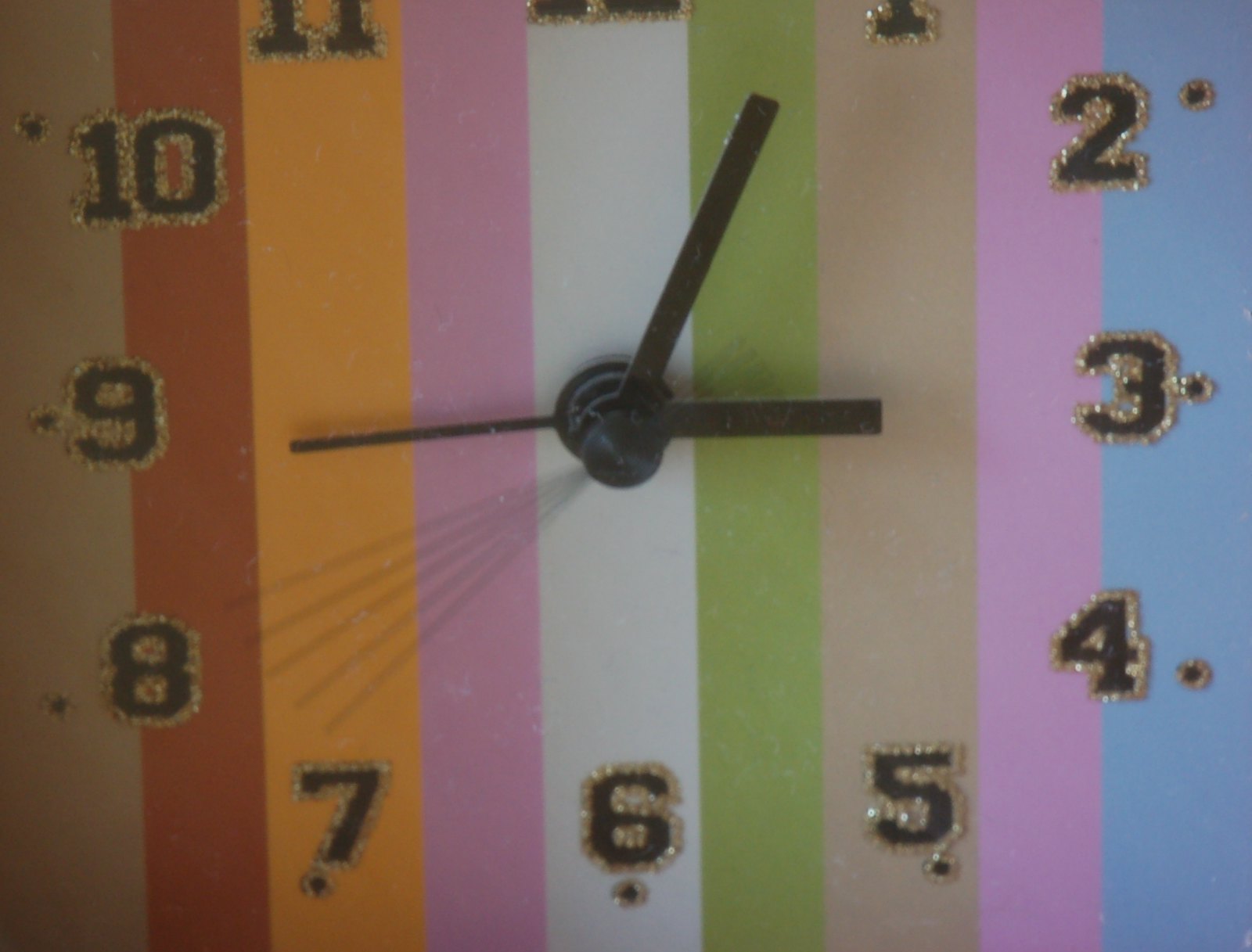The image is a close-up photograph of a vibrantly striped clock face, featuring vertical stripes in an array of colors, including brown, red, orange, pink, white, green, tan, another pink, and blue. The black numbers 1 through 12 on the clock are outlined with gold glitter. Although not all numbers are fully visible due to the zoomed-in nature of the photo, the ones that can be seen include 2, 3, 4, 5, 6, 7, 8, 9, 10, with portions of 11 and the edges of 12 and 1 also visible. The clock hands—comprising a rectangular hour hand, a thinner minute hand, and an even thinner second hand—indicate the time is 3:05. The minute hand is either at the 5 or 1, the hour hand at the 3, and the second hand pointing to the 9. There is also a blurred shadow-like image suggesting motion, likely from the second hand. The central white stripe is where the clock hands are secured, acting as the focal point of the design.